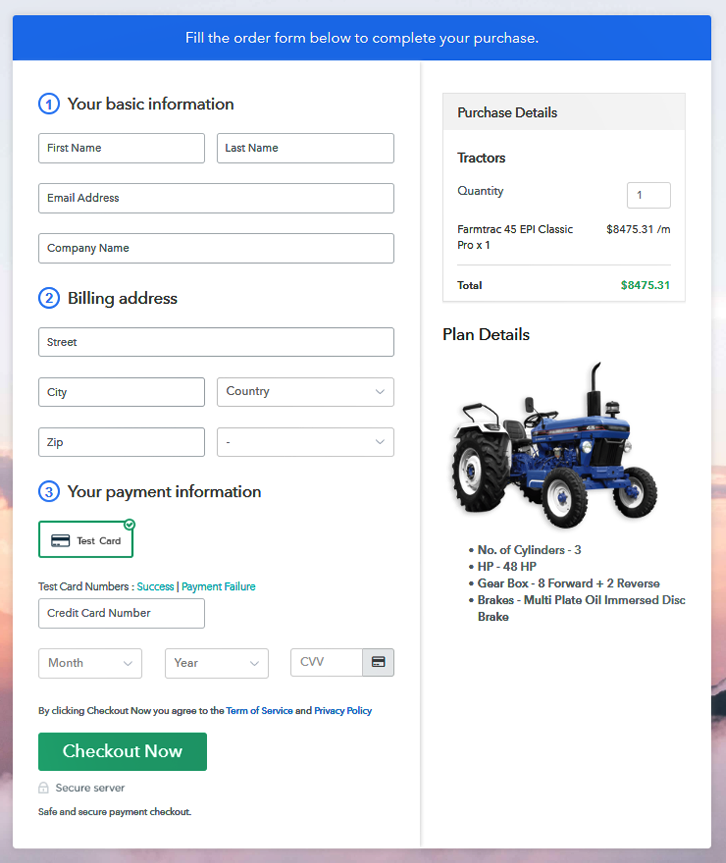The image depicts an online order form designed to complete a purchase. The top section prompts the user to fill in their basic information, which includes fields for first name, last name, email address, and company name. Following this, the user must provide their billing address, requiring details such as street address, city, country, zip code, and any additional address information.

Next, the form requests payment information, asking for the customer's card number, expiration month and year, and CVV code. On the right side of the form, purchase details are displayed. The user is purchasing a single unit of the "FarmTrack 45 EPI Classic Pro" tractor, priced at $8,475.31. 

An image of the tractor appears at the bottom of the form. The tractor is blue, featuring large rear wheels and smaller front wheels. Key specifications are highlighted: it has three cylinders, 48 horsepower (HP), and a gearbox with eight forward and two reverse gears. The tractor also features multi-plate oil-immersed disc brakes. The form assures that the checkout process is secure, giving customers peace of mind regarding the protection of their payment information.